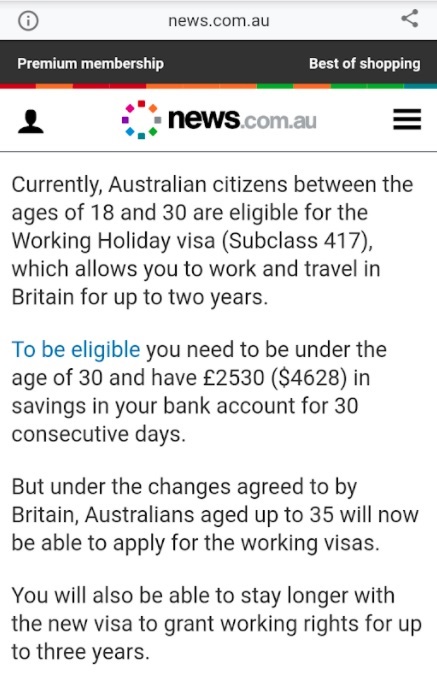**On a white background of the webpage, there is a light gray border at the top that spans across the page. Within the gray border, there is a gray-outlined circle featuring a gray eye. Adjacent to this circle, the text "news.com.au" is displayed in black. Below this, a dark gray border appears. On the left side of this border, the white text reads "Premium Membership," followed by the words "Best of Shopping" underneath. Beneath this, "news" is in black, with ".com.au" in gray accompanied by three black lines. A thin black line runs underneath this text. The main content in black reads: "Currently, Australian citizens between the ages of 18 and 30 are eligible for the worker's holiday visa (subclass 417), allowing them to work and travel in Britain for up to two years." The next paragraph starts with "To be eligible" in blue, then continues in black: "you need to be under the age of 30 and have €2,530 (approximately $4,628) in savings in your account for 30 consecutive days." The text then notes: "Under the changes agreed to by Britain, Australians aged up to 35 will now be able to apply for the working visas, with the new visas granting working rights for up to three years."